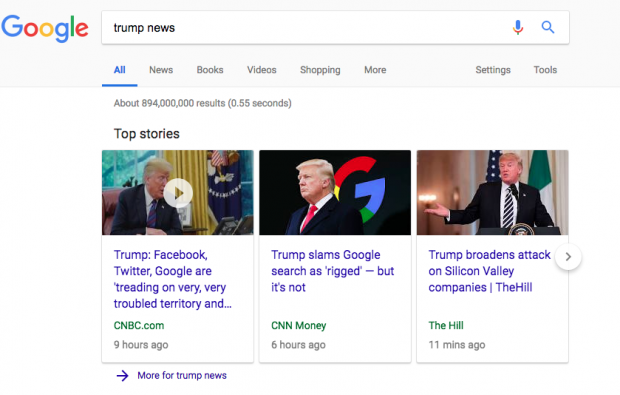This is a detailed screenshot of a Google search results page. At the top, there's a wide, light gray banner that is almost white. In the upper left-hand corner, the colorful Google logo is prominently displayed. Centered at the top of the page is a long search bar containing the query "Trump News." To the right of the search bar are a microphone icon and a magnifying glass icon signifying voice search and search functions, respectively. Beneath the search bar, a horizontal line of menu options is visible. The first menu option is highlighted in blue and underlined, labeled "All." The remaining options—displayed in gray—are "News," "Books," "Videos," "Shopping," "More," "Settings," and "Tools." 

The search results indicate approximately 894 million results found in 0.55 seconds. Directly below these details, the "Top Stories" section is displayed featuring three horizontally aligned articles with thumbnails, all pertaining to Donald Trump. The article on the left, from CNBC.com, is titled "Trump: Facebook, Twitter, Google are treading on very, very troubled territory" and was posted nine hours ago. The center article, from CNN Money, is headlined "Trump slams Google search as rigged, but it's not" and was posted six hours ago. The right-most article, from The Hill, reads "Trump broadens attack on Silicon Valley companies" and was posted 11 minutes ago.